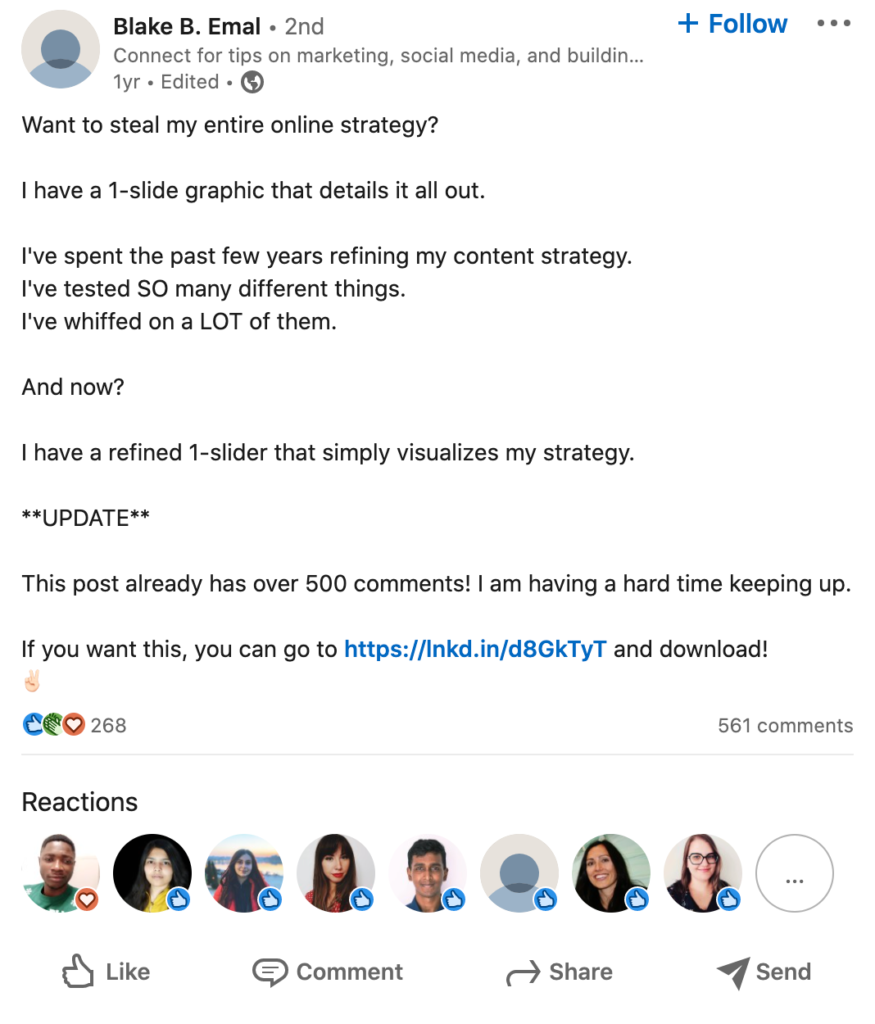**LinkedIn Post by Blake B. Email**

Profile Details:
- **Profile Image:** Generic icon depicting a cartoon person, represented by two circles (one for the head and a partial one for the body).
- **Username:** Blake B Email
- **Bio:** "Connect for tips on marketing, social media, and building..." (Note: Bio truncated).
- **Account Duration:** 1 year
- **Follow Option:** Available (blue "Follow" button with a plus sign)
- **Post Edit Status:** Edited

**Post Content:**

"Want to steal my entire online strategy? I have one slide graphic that details it all out. I've spent the past few years refining my content strategy. I've tested SO many different things. I've whiffed on a LOT of them. And now?  
I have a refined one-slider that simply visualizes my strategy.

**⭐️⭐️UPDATE⭐️⭐️**
This post already has over 500 comments! I'm having a hard time keeping up. If you want this, you can go to [LinkedIn link] and download it."

**Engagement Statistics:**
- **Reactions:** 268
  - Thumbs up
  - Love
  - Clapping hands
- **Comments:** 561

**Interactive Icons:**
- **Reactions Summary:** Displaying icons of 8 users, followed by a "more" indicator.
- **Post Interaction Options:**
  - Like
  - Comment
  - Share
  - Send